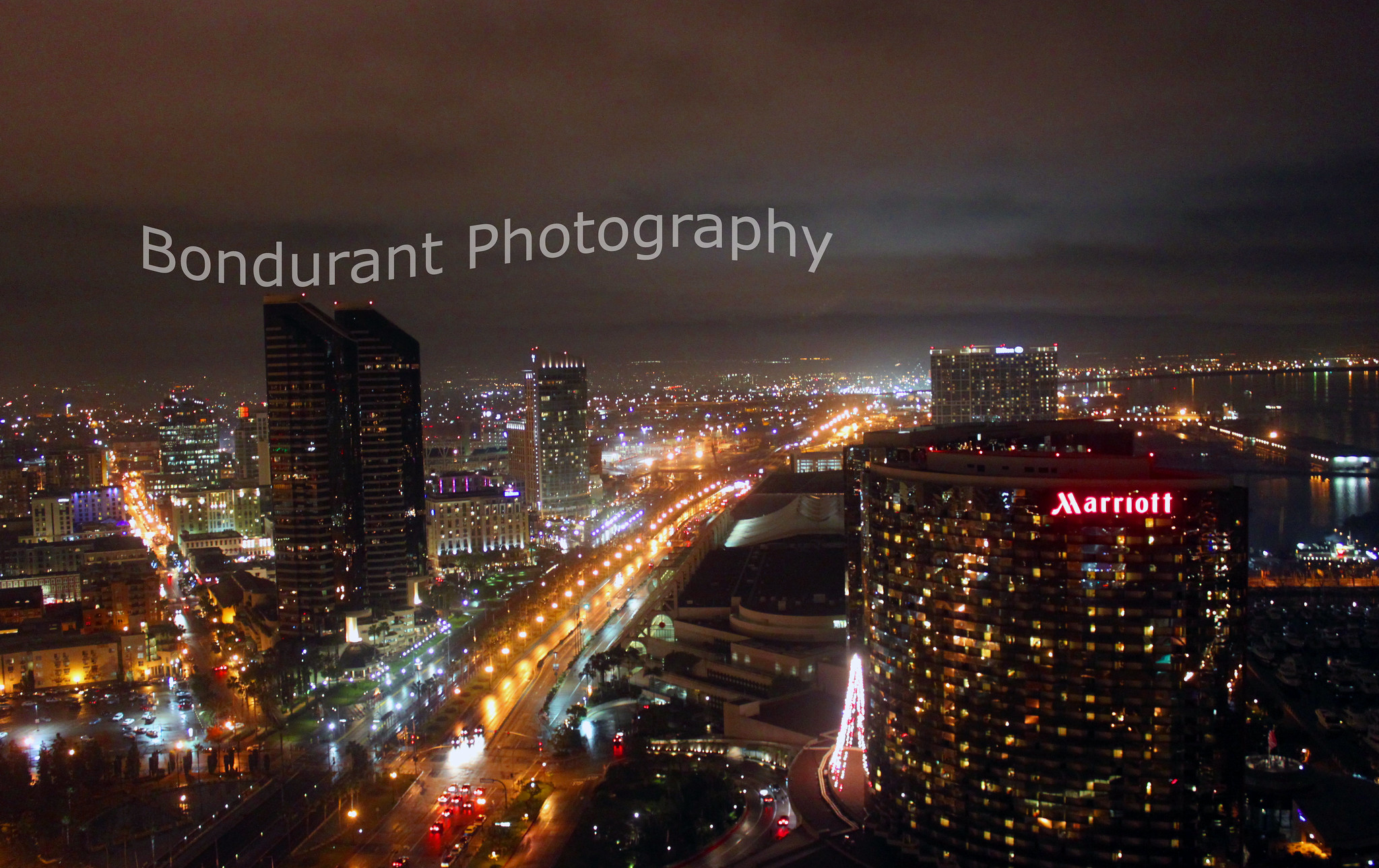This richly detailed nighttime aerial photograph captures a bustling city skyline illuminated under a cloudy sky. The city lights create a radiant glow that reaches up to the clouds, casting an enchanting sheen over the entire scene. Dominating the image, high-rise buildings are dotted along the horizon, including the distinct Marriott Hotel on the right-hand side, easily recognizable by its semicircular structure and red "Marriott" signage atop. The building is approximately 25 stories tall, with many of its rooms brightly lit.

The composition is punctuated by a major road running through the center, its path lit by a series of glowing streetlights and flanked by smaller city buildings ranging from 15 to 20 stories tall. Another road diverts from the main thoroughfare towards the top left of the frame. On the left side, two buildings of equal height stand out among the traditional cityscape. Towards the bottom right, beyond the Marriott, a glimpse of water can be seen, adding depth to the urban setting. 

A subtle watermark, "Bondurant Photography," is imprinted in the top left corner, accrediting the creator of this captivating cityscape.

A few cars can be spotted navigating the streets, adding a sense of movement and life to this serene urban tapestry.